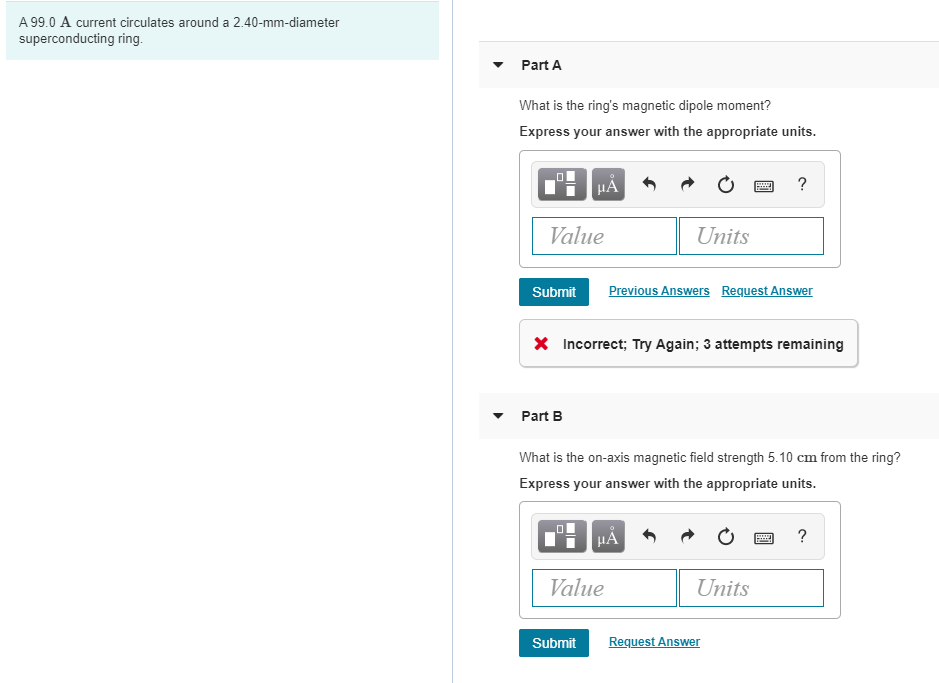The image depicts an interface with a clean white background, organized into two vertically separated columns by a thin pale blue line. 

In the left column, at the top, there is a decorative light blue ribbon. Just below the ribbon, black text reads: "99.0 A current circulates around a 2.40-mm-diameter superconducting ring."

In the right column, the top portion features a light gray banner with black text that reads "Part A" alongside a downward arrow symbol. Below this banner, black text asks the question: "What is the ring's magnetic dipole moment? Express your answer with appropriate results."

Beneath the question, there is a rectangular input area with two gray boxes. The first box, labeled "Value," is intended for numerical input, while the second, labeled "Units," is for specifying the measurement units. Below these input fields, a clickable blue box labeled "Submit" is positioned to process the answer. 

Adjacent to the submission area are two options: "Previous Answers" and "Request Answer." Below these options, another rectangular gray box contains a red "X" icon and black text stating: "Incorrect. Try again." This section also notes there are "Three attempts remaining."

Further down, another light gray banner labeled "Part B" with a downward arrow is displayed. This section mirrors the layout of Part A, with boxes for value and units, alongside a blue submit button.

Additionally, there is a blue box at the bottom posing the repeated question: "What is the ring's magnetic dipole moment?"